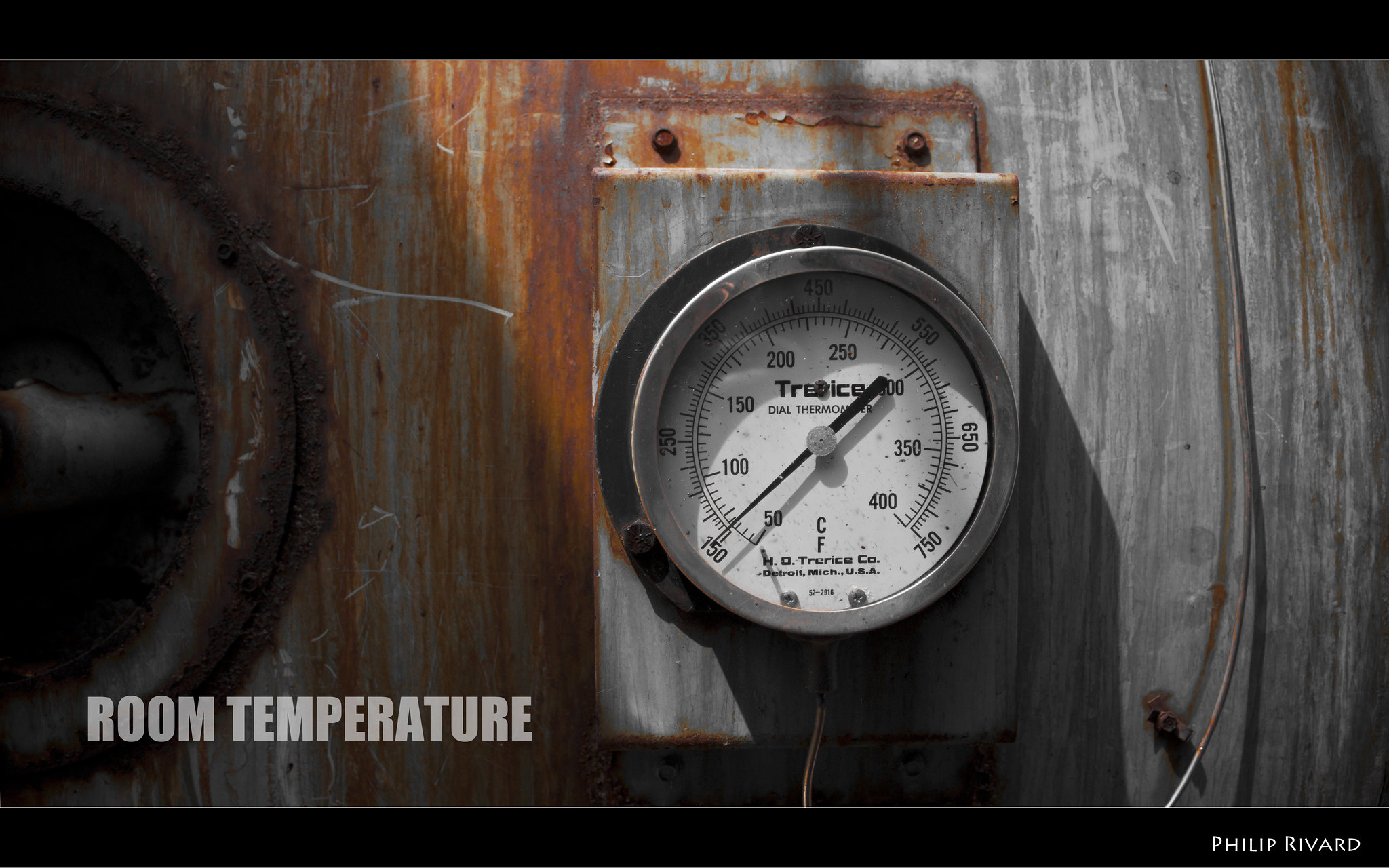The photograph depicts an indoor setting featuring a detailed gauge. The gauge, predominantly black and white, is encased in a silver frame and mounted against a silver, rusty surface. The exterior of the gauge is marked with increments, reading 150, 250, 350, 450, 550, 650, and 750. The inner markings of the gauge indicate finer measurements of 50, 100, 150, 200, 250, 300, 350, and 400. The needle of the gauge points towards the lower left-hand corner at the 150 mark. Centrally, the gauge displays the word "Trevis." In the lower left-hand corner of the image, “Room Temperature” is written in gray text, and in the lower right-hand corner, the name “Philip Rivard” is inscribed. The photograph is rendered in a square rectangular format, capturing every intricate detail of the gauge and its surroundings.